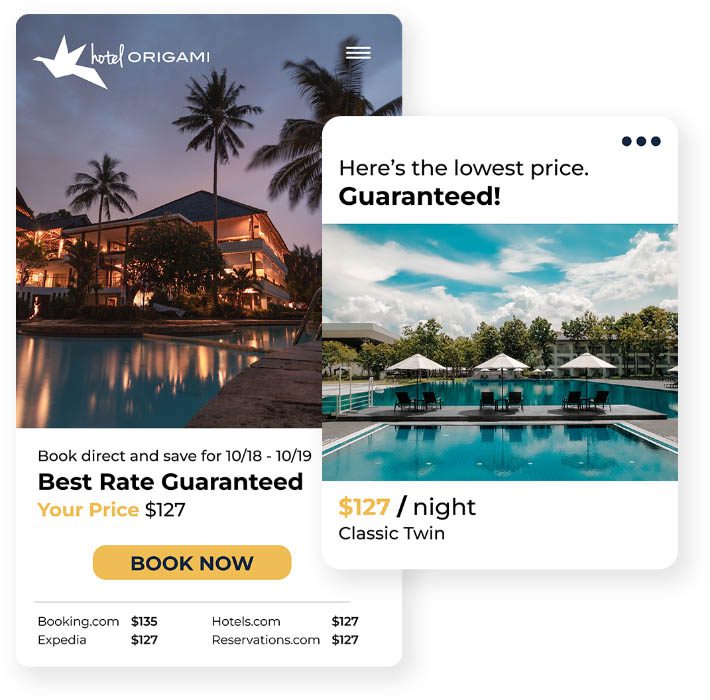The visual consists of two images arranged vertically, with one smaller image positioned over the larger image on the left and to the right side. The larger image prominently displays a logo featuring what appears to be an origami crane, with "Hotel Origami" written in white text. In the top right corner of this image is a three-horizontal-bars icon, commonly known as the hamburger menu.

To the right of the larger image is a picture depicting a luxurious tropical hotel setting, showcasing abundant water features, palm trees, and open, well-lit areas. The text overlay on this image advertises a special offer: "Book Direct and Save for October 18th to October 19th. Best Rate Guaranteed." The price is listed as $127 per night, with a call-to-action button encouraging viewers to "Book Now." Additionally, a price comparison is provided with rates from various booking platforms: Booking.com at $135, Hotels.com, Expedia, and Reservations.com each at $127.

A pop-up section further emphasizes "Here's the Lowest Price Guaranteed," accompanied by a three-horizontal-dots icon for additional information. This smaller overlay image appears to be another view of the Hotel Origami, highlighting multiple pools and lounge areas, with a rate of $127 per night for a classic twin room. The images and information suggest that this content is sourced from an online reservation platform or app, likely targeting potential guests looking for the best deals.